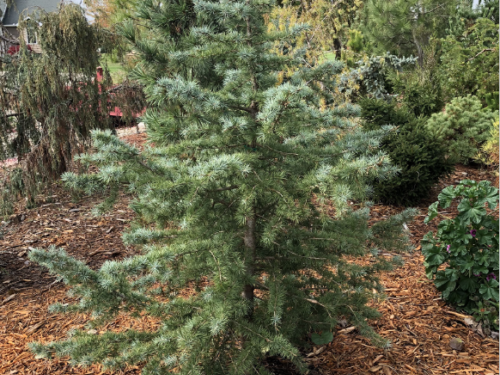The image depicts a daytime outdoor scene near a house, partially visible in the upper left corner. The house has brown siding, a gray roof, and a white-trimmed window. Dominating the center-right of the photo is a young evergreen or pine tree with a small trunk and horizontally extending branches. The ground below is covered in mulch and wood chips, indicating intentional planting by the homeowner. Surrounding the central tree are various small plants and bushes, typical of a nursery's offerings. There is also a hint of blue sky in the upper right corner, adding to the daytime ambiance. To the left of the tree, closer to the center, there's an indistinct red object that might be a vehicle. The image overall features a landscaped, garden-like space with a mix of young trees and shrubbery, suggesting a well-tended but somewhat cluttered area.